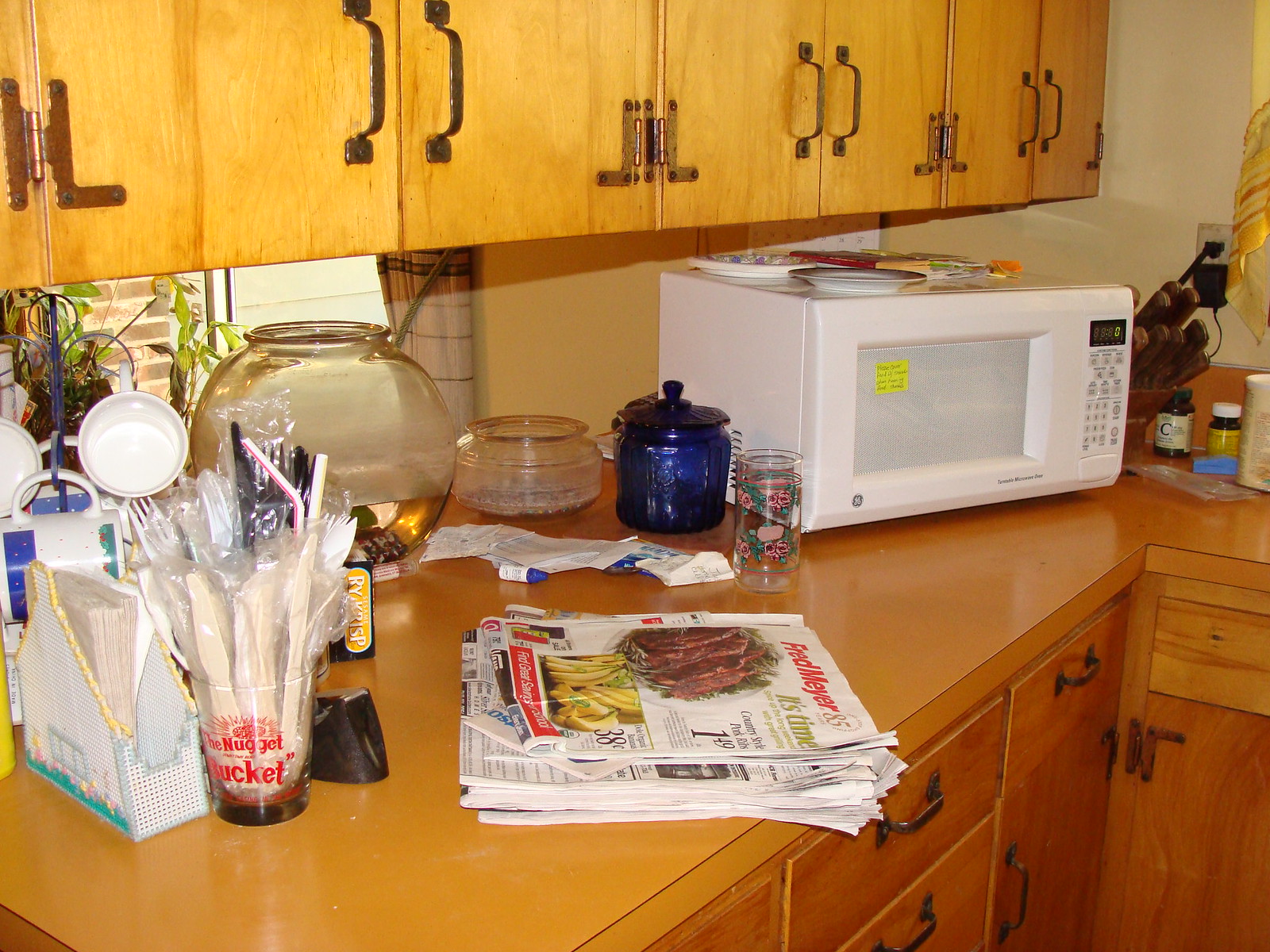This detailed photograph captures a well-used kitchen countertop, showcasing a blend of functionality and homey warmth. The countertop, L-shaped and a light brown laminate, provides ample workspace. It is complemented by medium brown wood cabinets below, adorned with dark metal handles, creating a cohesive look with the upper cabinets, which are in the same light brown wood and feature identical dark metal handles.

On the left edge of the countertop lies a newspaper, prominently featuring an advertisement for "Fred Meyer 85." Near the newspaper, a plastic cup branded with "The Nugget Bucket" in red letters holds several pieces of plastic silverware. Towards the back of the countertop, a round fishbowl sits partially filled with water, adding a touch of life to the scene.

On the right side of the countertop, a white microwave stands, topped with a few plates. Next to the microwave is a knife block, housing several knives, indicating a well-prepared kitchen space ready for meal preparation.